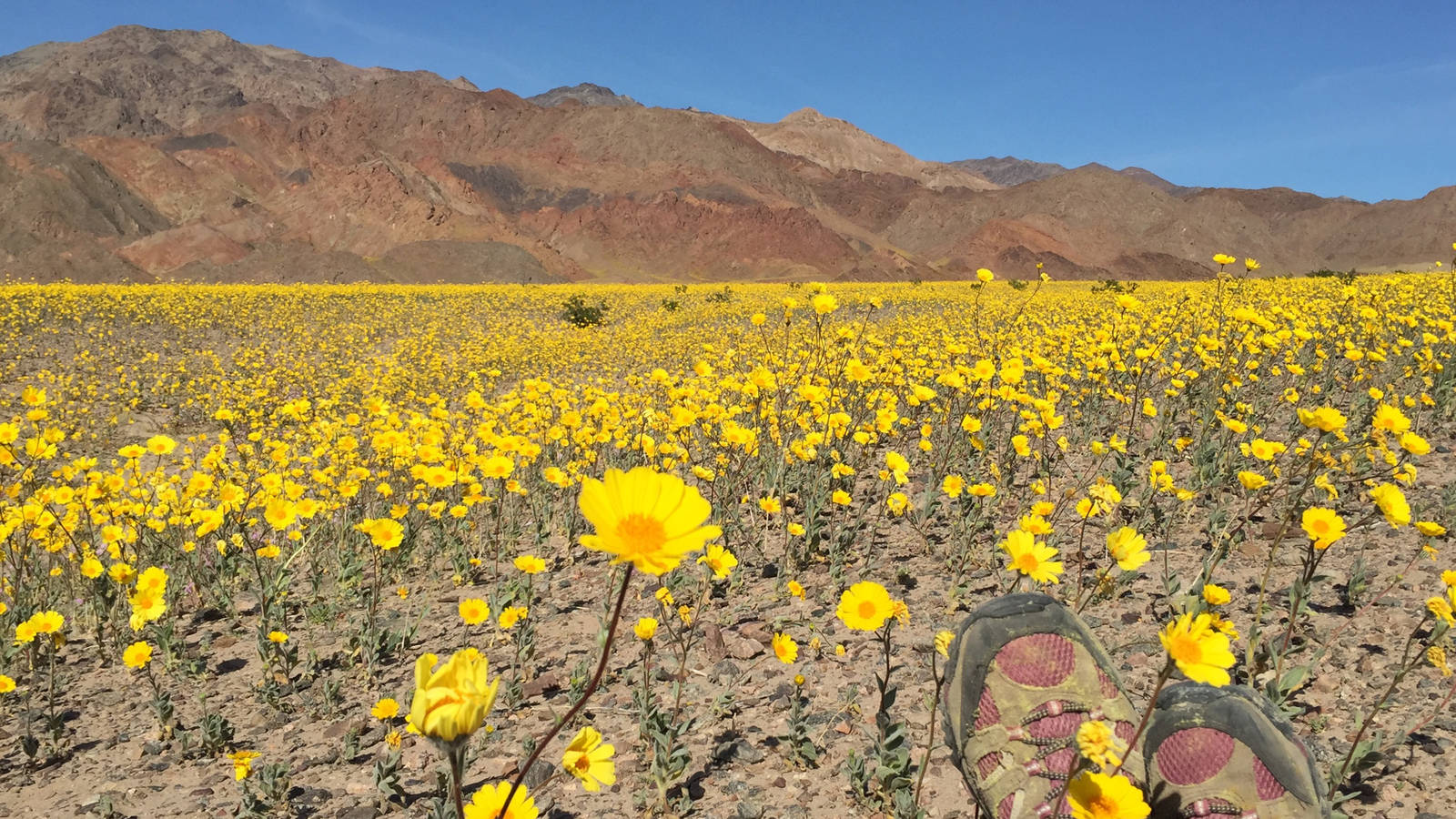The photograph depicts a vibrant field of yellow flowers with orange centers, thriving in a flat, brown dirt landscape. The flowers, reminiscent of Asteraceae, have relatively long, thin stems supporting their delicate blooms. In the bottom right corner of the image, a person’s crossed feet, clad in red and tan hiking shoes, are visible, suggesting the individual is sitting amidst this natural beauty. They appear to be enjoying a sunny, cloudless day that accentuates the vivid colors of the flowers. In the distance, a range of high, rugged mountains stretches across the background, displaying shades of copper, light brown, and gray, with the peaks ascending toward the left side of the image. The clarity of the blue sky further enhances the breathtaking and serene atmosphere of the scene.